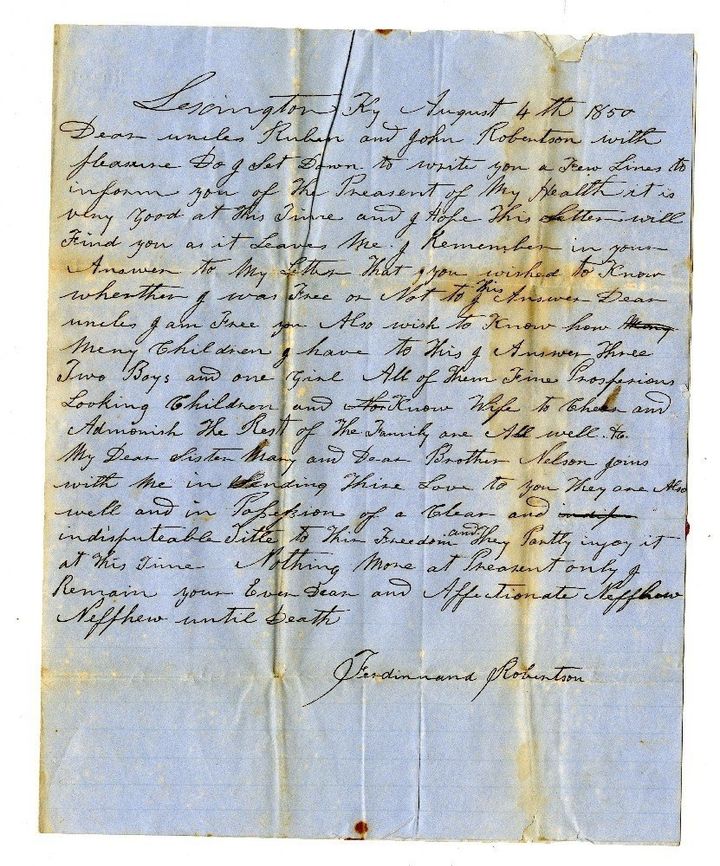The image depicts a rectangular photograph of an aged piece of paper, measuring approximately five inches in height and three to four inches in width, viewed from above. The paper features very faint horizontal lines and exhibits a gradient of gray tones—from a lighter shade at the bottom to a darker gray at the top, possibly due to shadowing or the paper’s natural aging process. Distinct creases and folds are evident, with yellow to light tan stains marking these folds, suggesting the paper had been folded multiple times. Notably, there are vertical stains running from the top left corner downwards, and two horizontal stains stretching from left to right, along with two additional vertical stains closer to the center and right side, indicating areas where the paper was folded.

The document contains a handwritten letter in black cursive ink, dated August 4th, 1850, and signed by someone who appears to be Ferdinand Robertson. The script is intricate and somewhat difficult to read, yet the date is clearly discernible. The paper itself, though aged and stained, retains distinct blue horizontal lines typical of lined paper. Additionally, a small red mark is visible at the bottom of the page, which could be a blood stain, rust stain, or some remnants of a staple, adding to its mysterious and historic character.